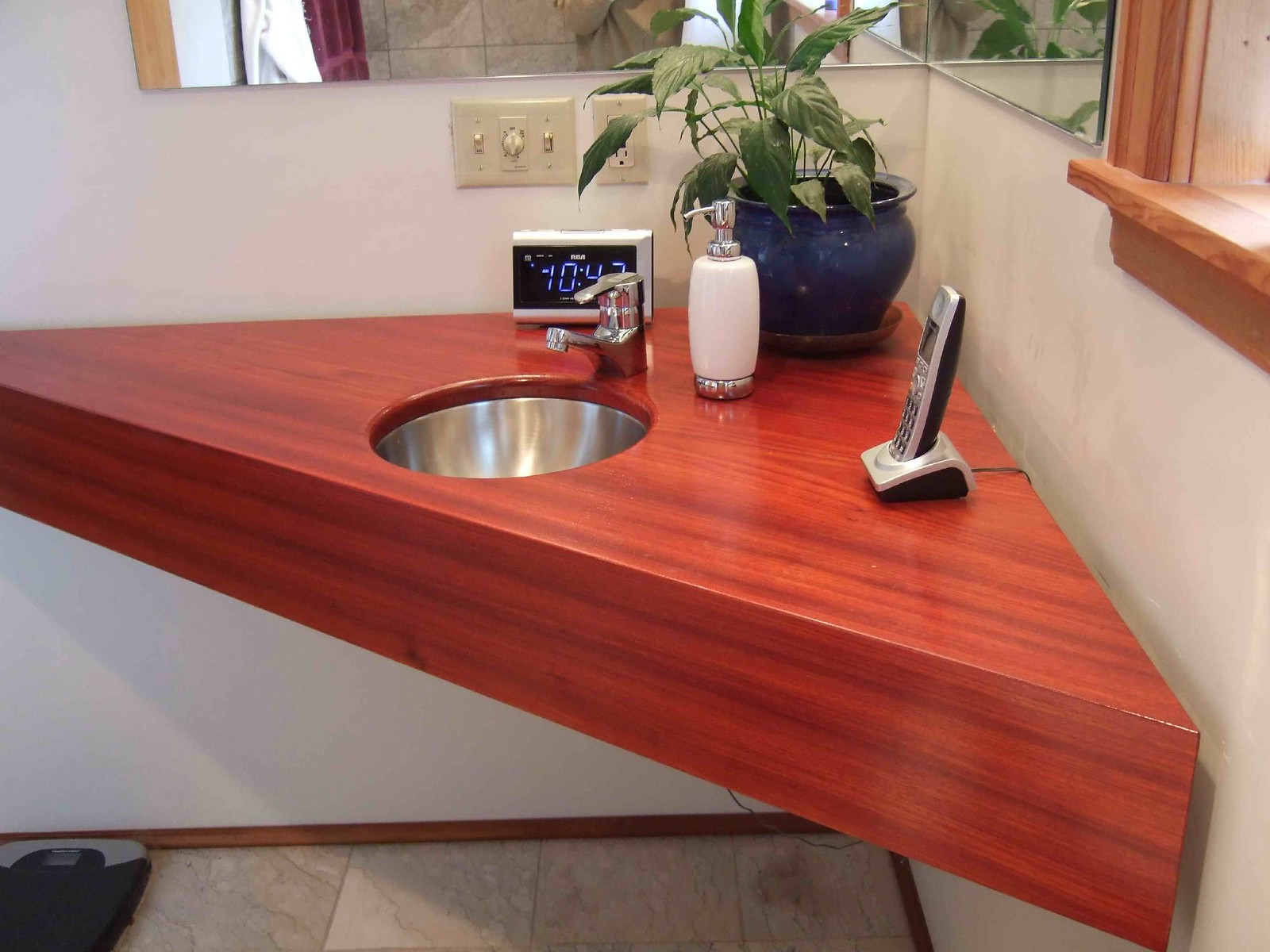The image captures a quaint corner sink area meticulously detailed. The flooring is adorned with brownish and whitish tiles, complementing the thin red wood baseboard skirting the walls. A dark grey and light grey weight scale is placed on the floor near the sink. The countertop is a striking reddish-brown with wood paneling featuring horizontal lines. 

The circular sink boasts a polished silver interior, and the accompanying tap is also silver. Adjacent to the sink is a white porcelain soap dispenser with a silver bottom, cap, and drip nozzle. On the counter's edge, a silver and black portable phone rests on its charger. Adding a touch of nature, a blue pot teeming with vibrant green leaves occupies a corner of the countertop.

Above the sink, a digital clock with a silver rim and black face displays the time, 10:47 AM, in light blue digits. The left side of the counter holds a yellow light fixture with a dimmer switch, while a yellow power outlet is installed to the right. High above, a mirror catches a partial reflection of the room, and a wooden-framed window peeks out from the top right corner, completing this detailed and cozy nook.